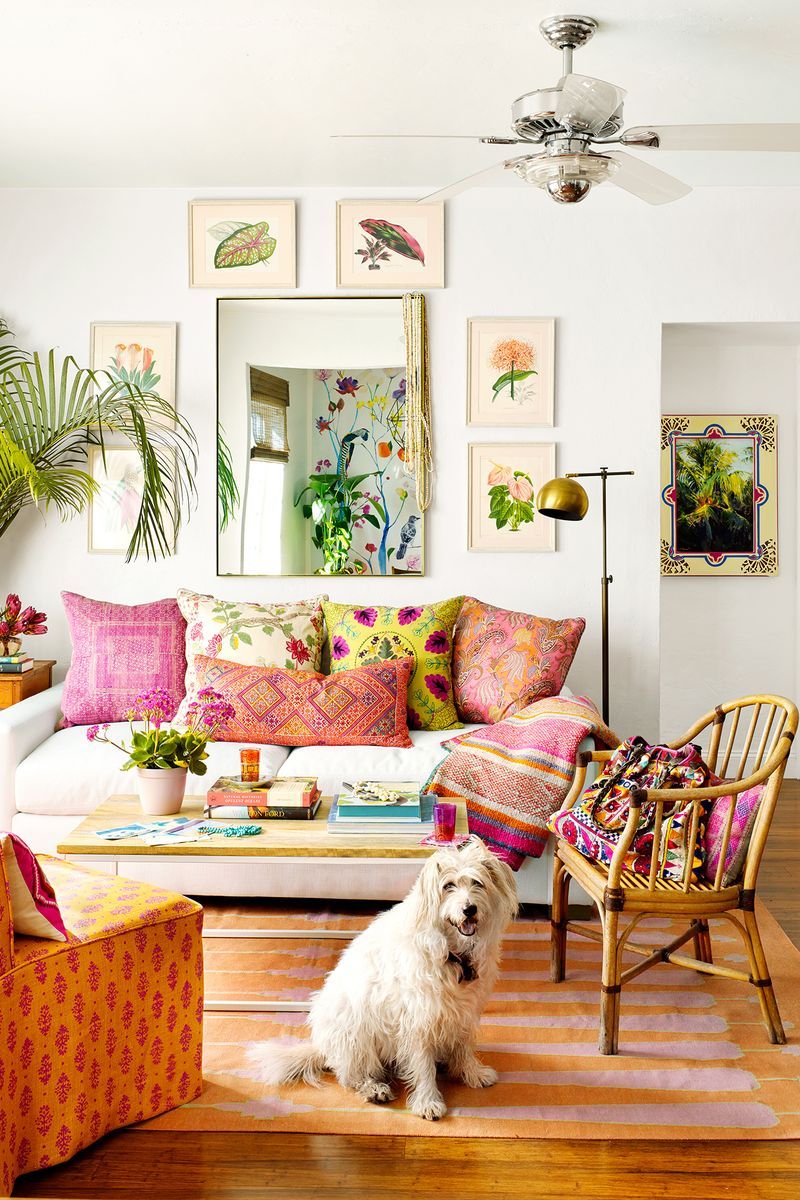This vertically oriented photograph captures a bright and inviting contemporary living room, characterized by its floral theme and cozy ambiance. The room features polished hardwood floors and an orange and purplish striped rug that adds a pop of color. Central to the image is a white, plush two-seater sofa adorned with a variety of throw pillows: pink and orange-hued pillows on either end, green floral-patterned cushions with red leaf designs in the center, and a long orange lumbar pillow in the front.

The back wall, painted in a cream color, prominently displays a vertical mirror flanked by six artistic representations of various plants arranged in a harmonious pattern, each with beige backgrounds. An additional medium-sized framed painting depicting nature is positioned toward the right side of the wall. There is also a ficus plant barely in frame on the upper left.

Above, the white ceiling hosts a metal-structured ceiling fan with white blades. A gold floor lamp with a pole and a half-circle fixture illuminates the right side of the sofa, enhancing the room's warm atmosphere.

In front of the sofa, a light wood coffee table accessorized with a potted plant, a book, and coasters serves as a focal point. A white shaggy sheepdog sits on its hind legs directly in front of the coffee table, gazing endearingly at the camera.

To the right of the dog is a wicker chair with a bentwood arched back, furnished with additional throw pillows. To the left of the shaggy dog and facing the sofa, there is a plush armchair upholstered in an orange-yellow floral pattern.

Overall, the room is a well-curated space that exudes a welcoming and stylish vibe, perfect for relaxation and comfort.